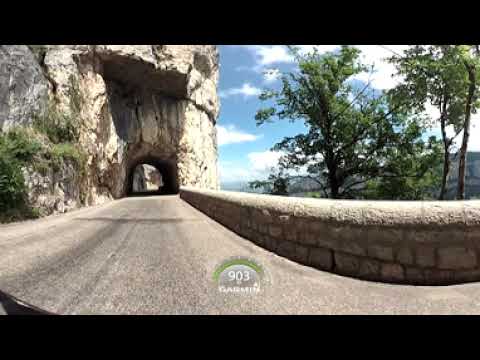This panoramic picture, taken from inside a car in broad daylight, captures a narrow, gravel two-lane road winding along the side of a mountain. To the left of the road is a sheer rock cliff that extends directly into the roadway, while to the right is a stone railing beside a plunging 3,000-foot drop into a lush, tree-filled valley. The stone grey ledge and concrete curve top barrier curve gracefully along the road, highlighted by some panoramic distortion. The road itself shows signs of previous travel with visible tire tracks. Above the scene, the sky is a clear, light blue adorned with bright white clouds. At the bottom center of the image, there is a green Garmin dial displaying '903' with some additional, partially illegible text. The upper part of the mountain features trees and various plants, enhancing the rugged, natural beauty of the landscape. In the distance, beyond the valley, another towering rock cliff rises, forming a dramatic backdrop to the serene yet precarious roadway.